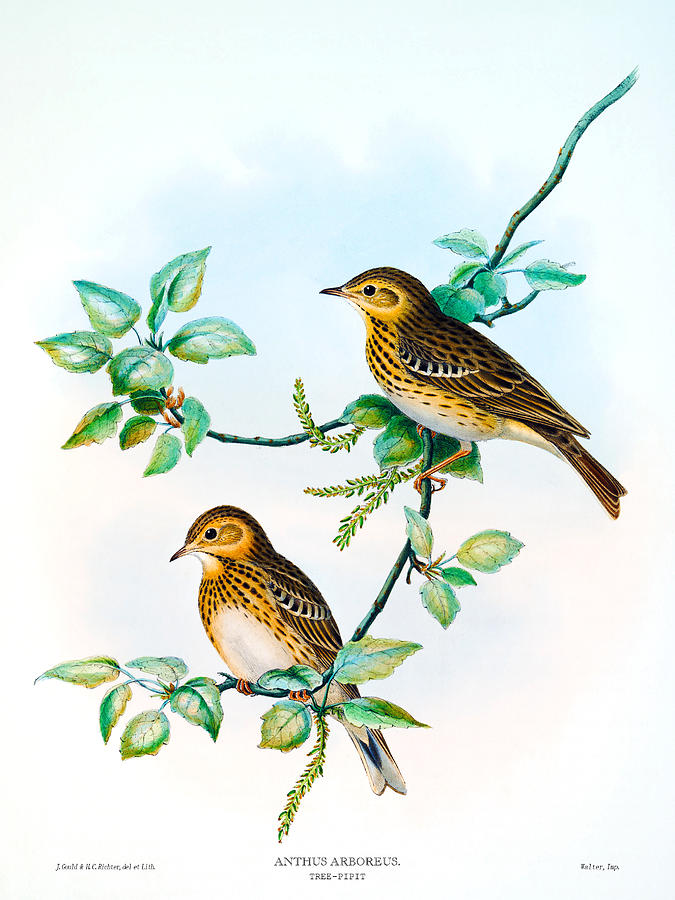The image is a vertically oriented, hand-drawn or digitally created poster with no borders, featuring a nature scene on a bluish-white background that gradually transitions to gray clouds in the middle. Dominating the composition, a branch starts at the bottom middle, extending upward to the upper right, adorned with light green leaves that become larger and more abundant as they ascend. Perched on this branch are two identical birds, positioned vertically with one above the other, both facing left. These birds have white undersides, small black beady eyes, and yellow and brown bodies with brown spotting on the yellow areas. Their feet are clearly visible, gripping the branch, along with their wings, beaks, and tails. Subtle yet intricate details mark their feathers, adding to the lifelike portrayal. The background is predominantly white, with some text in light-colored, unreadable font below the scene.